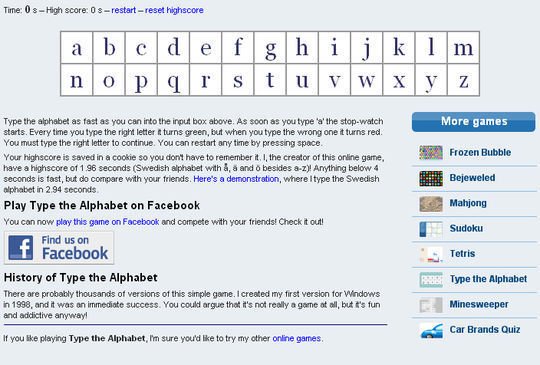This image has a distinctly nostalgic feel, reminiscent of mid-2000s internet designs. The primary background is a very light blue that immediately draws the eye to a prominent grid in the center. This grid is split into two horizontal rows, with the alphabet arranged sequentially in white-backed cells: A through Z divided between the rows. 

At the top, black text displays both "Time: 0 seconds" and "High Score: 0 seconds," indicating a game is in progress. There are blue hyperlinks beneath these readings that say "Restart" and "Reset High Score." Just below, a descriptive box explains the game's objective and rules. 

Underneath this description, there’s a banner prompting users to "Find us on Facebook," adorned with an older version of the Facebook logo, which is clickable. To the right, another blue banner with white text offers links to "More Games." This section lists eight web-based minigames, including Tetris, Bejeweled, Frozen Bubble, and Minesweeper.

The game challenges users to type the alphabet as quickly as possible into an input box at the top. The timer starts as soon as the letter 'A' is typed. Correctly typed letters turn green, while mistakes turn red, forcing the player to retype the correct letter to proceed. The spacebar can be used to restart the game at any point. Additionally, a detailed scoring explanation follows, ending with a blue hyperlink for a demonstration, offering further context for new players.